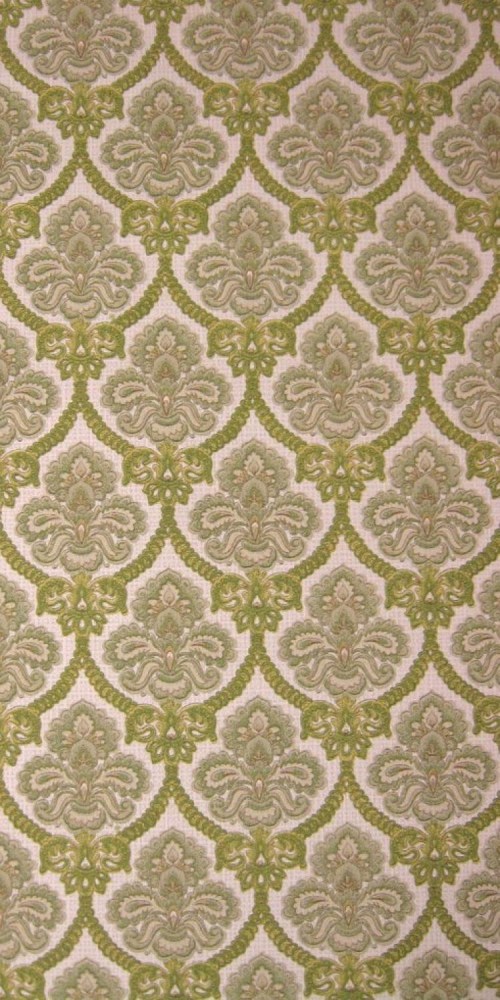The image features a vertically aligned rectangular piece of fabric, possibly upholstery or wallpaper, showcasing a repeating pattern. The background is a light tan color with a greenish-gold, almost olive, intricate floral and paisley design. The pattern consists of rows of paisley shapes, which alternate in a staggered fashion, forming diagonal lines across the fabric. Each paisley shape is outlined by a textured, squiggly rope-like detail. This detailed and seamless arrangement includes hues of green, light brown, tan, and a hint of pink or yellow, creating a visually appealing and harmonious design.